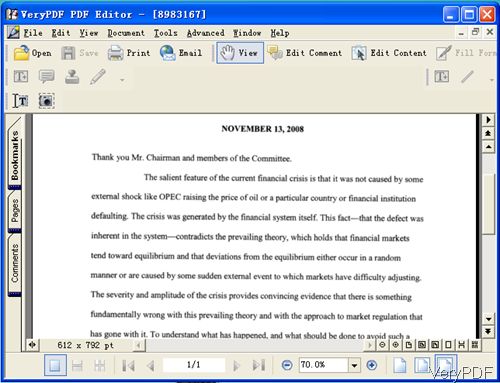The image displays a screenshot of an old computer operating system, resembling the Windows XP interface, viewing a PDF document within a PDF editor application called VeryPDF. The top window bar is blue with the typical 'X' close button found in Windows XP. The main toolbar shows options like File, Edit, View, Document, and Tools, alongside the VeryPDF identification number 8983167 in brackets. The text on the screen is a full-page PDF document dated November 13, 2008, addressing "Mr. Chairman and members of the committee" in bold black text at the top. The document, which appears in Times New Roman font, discusses the financial crisis and the inherent issues within the financial system, having decent paragraph spacing and margins. The left side of the screen features tabs labeled Comments, Pages, and Bookmarks. The bottom of the screen shows various status indicators, such as "612 x 792 PT" and "1-to-1 70.0%." The image features a muted color palette, predominantly blue, light blue, black, white, and gray, reminiscent of an older digital interface.